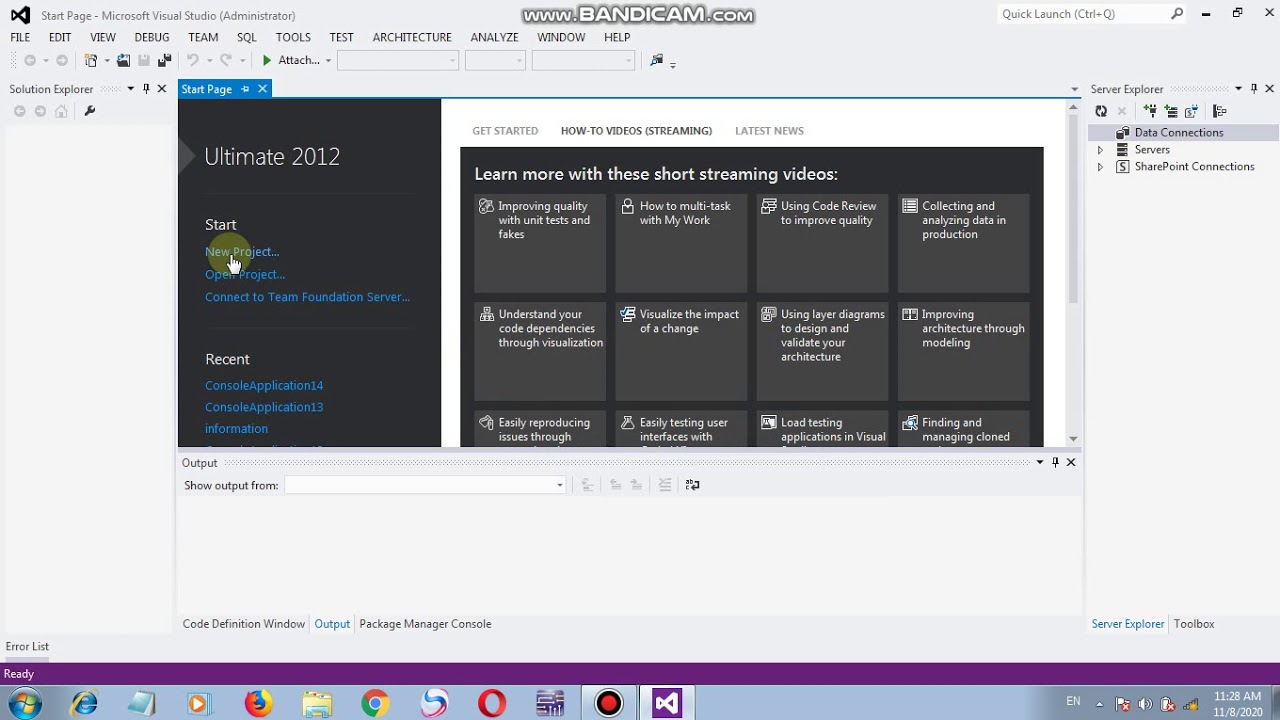Screenshot of the Microsoft Visual Studio website being viewed with administrator privileges. The top-left corner displays the title "Microsoft Visual Studio (Administrator)." Below the title are various menu tabs, including File, Edit, View, Debug, Team, SQL, Tools, Test, Architecture, Analyze, Window, and Help. At the top of the screen is a watermark that reads "www.bandicam.com," indicating that the image is likely a screenshot from a recording. This is further evidenced by an icon on the taskbar featuring a red dot, signifying active recording. The screenshot also captures the mouse cursor with a yellow highlight to indicate its position at the time of capture. Just above the cursor, the text "Ultimate 2012" is visible along with options to "Start New Project," "Open Project," and "Connect to Team Foundation Server."